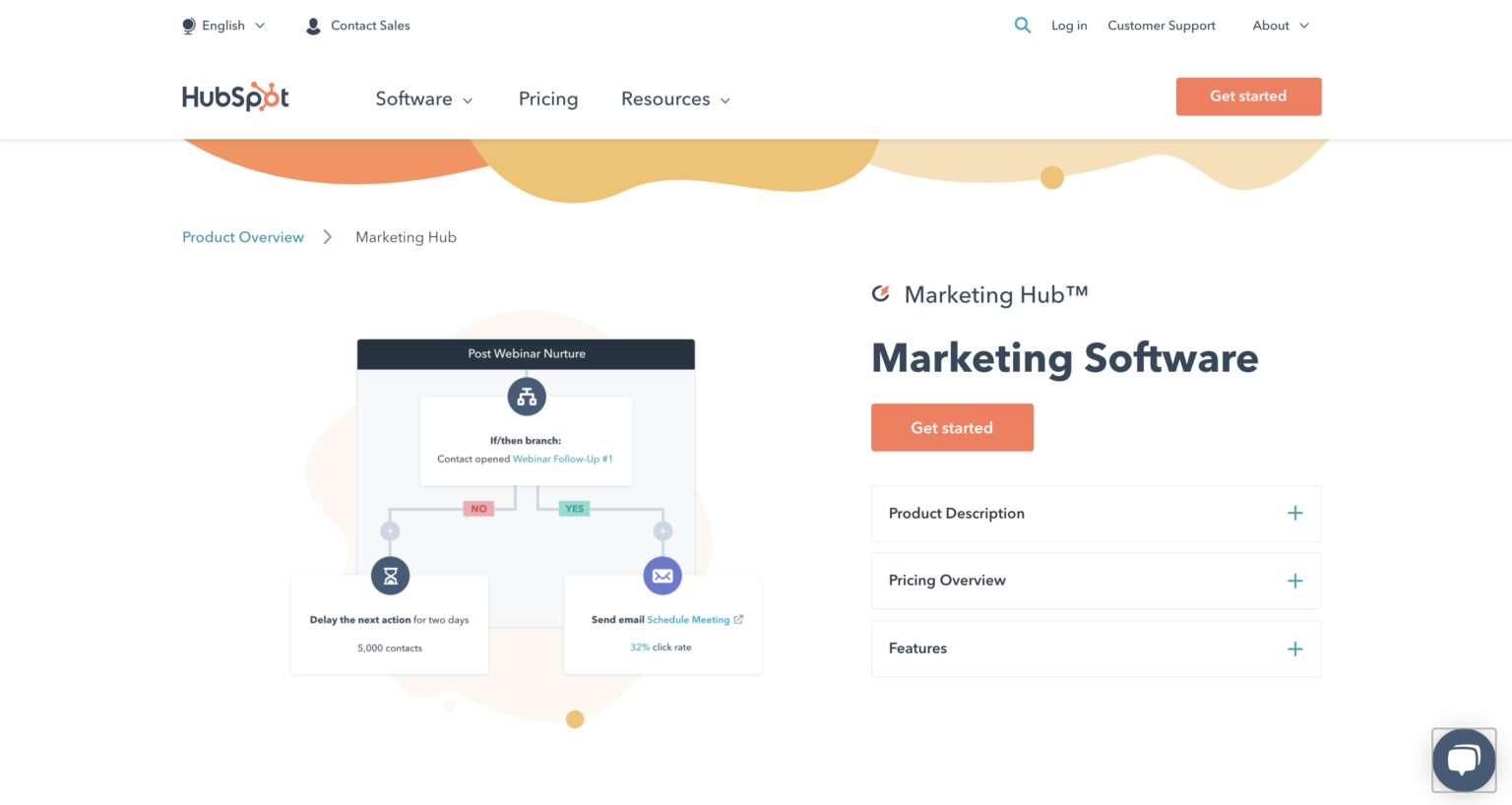In this comprehensive HubSpot screenshot, we observe the homepage of the HubSpot website. In the upper left corner, the language is set to English, followed by the labels "Content" and "Sales." Directly below this section resides the HubSpot logo, where all letters are black except for the "O," which features an orange design resembling a DNA atom.

To the right of the logo, three navigation categories are listed in gray text: "Software," "Pricing," and "Resources." In the upper right corner, there are several options, including a search bar, login option, customer support, and an "About" section.

An eye-catching orange rectangle just below these options prompts users to "Get Started." The primary background of the page is white. However, a splash of color draws attention in the lower section: an orange hue on the left, transitioning to a gold shade in the middle, and a pink tint on the right, with a small, orangish-brown circular element.

Further down on the right side of the screen, text lists various sections: "Marketing Hub," "Marketing Software," "Get Started," "Product Description," "Pricing Overview," and "Features." Below this list, there are three options in black text, each accompanied by a blue plus sign to the right.

The left side of the screen features a diagram with a light gray background. At the top of this diagram is a black header with text that appears to read "Post Webinar Nature," albeit in very small, hard-to-read font. This section, like the rest of the page, also resides on a white background.